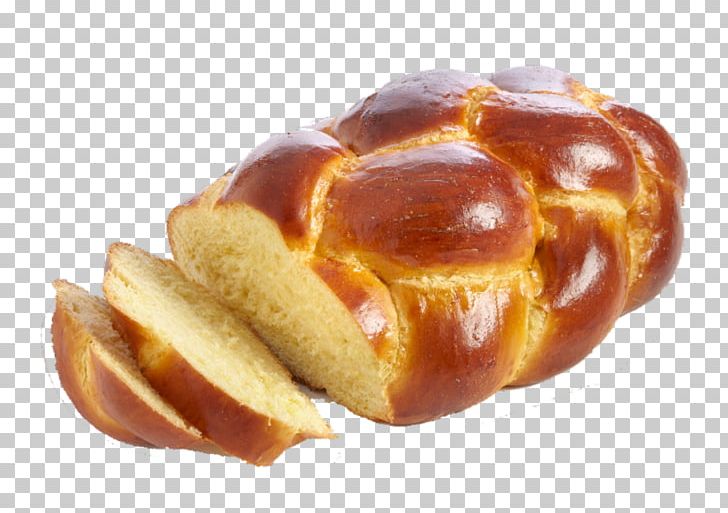The image features a beautifully-braided loaf of challah bread, renowned for its knotted design and rich egg-enriched dough. The loaf boasts a rich amber brown exterior, likely achieved with an egg wash, that contrasts strikingly with the soft, spongy pale yellow interior. Two slices have been partially cut from the loaf, revealing its fluffy texture and the characteristic yellow hue from the egg yolks. The braided top appears shiny, while the intricate braiding is highlighted with yellow lines between the braid marks. The loaf lies flat against a simple gray and white checkerboard background, emphasizing its artisanal quality and inviting texture.